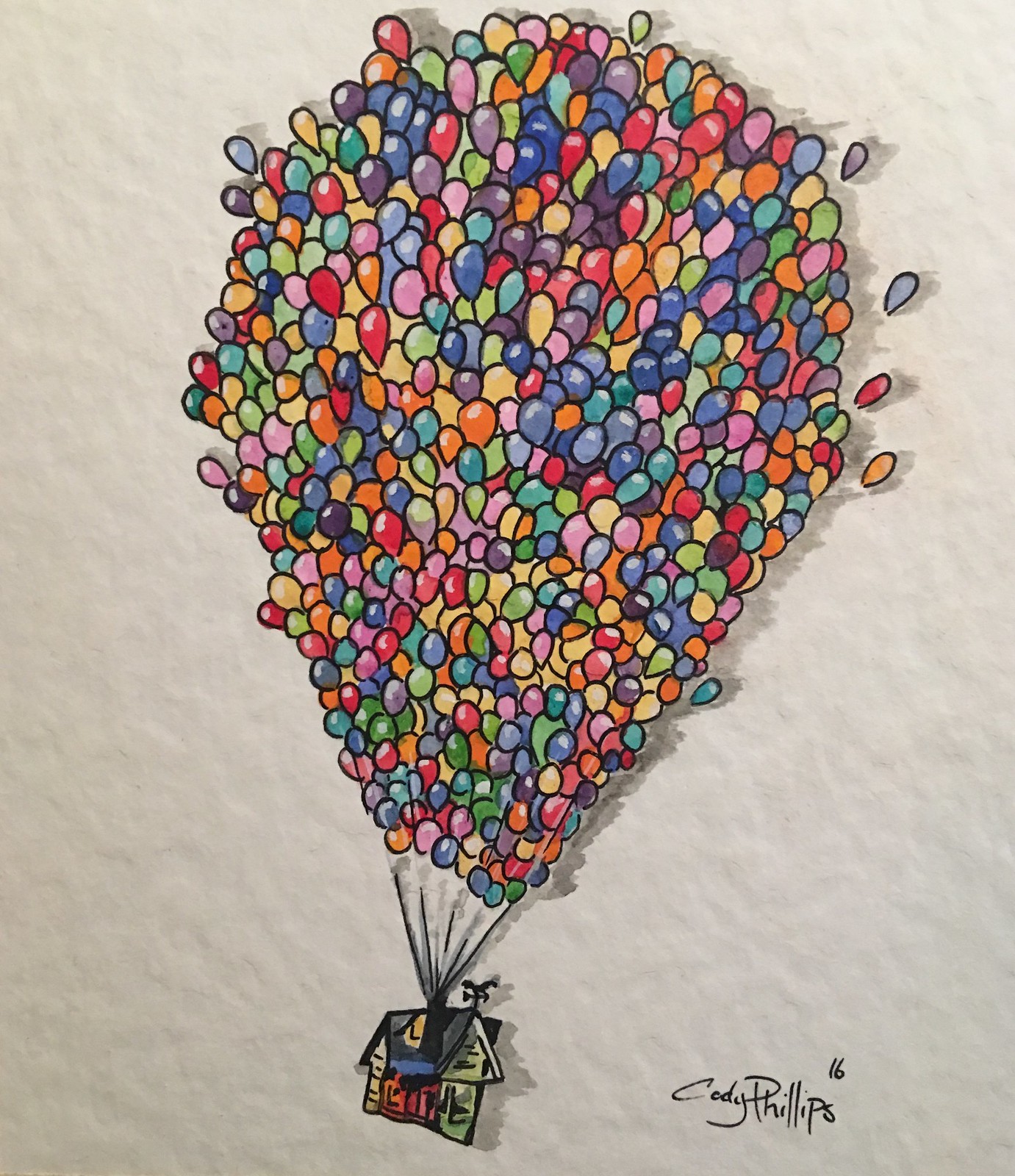The image resembles a detailed painting on textured, distressed ecru off-white paper. It features the signature of the artist, Cody Phillips, with the year '16' written above the "PS" in Phillips in black ink, located at the lower right corner. Dominating the composition are countless multicolored balloons in various shades of pink, blue, yellow, red, orange, purple, green, and more, taking up approximately three-quarters of the image. These balloons, in assorted rainbow colors, are attached to a small house situated at the very bottom one-sixth of the image. The modest house, adorned in red, yellow, blue, black, and green, is being lifted by the balloons, reminiscent of the iconic scene from the animated film "Up." The house features a weather vane on top, adding to its quaint charm. The striking contrast between the vibrantly colored balloons and the textured paper amplifies the whimsical and fantastical nature of the artwork. Shadows of both the house and the balloons can be seen in the background, giving the image depth and a sense of motion.